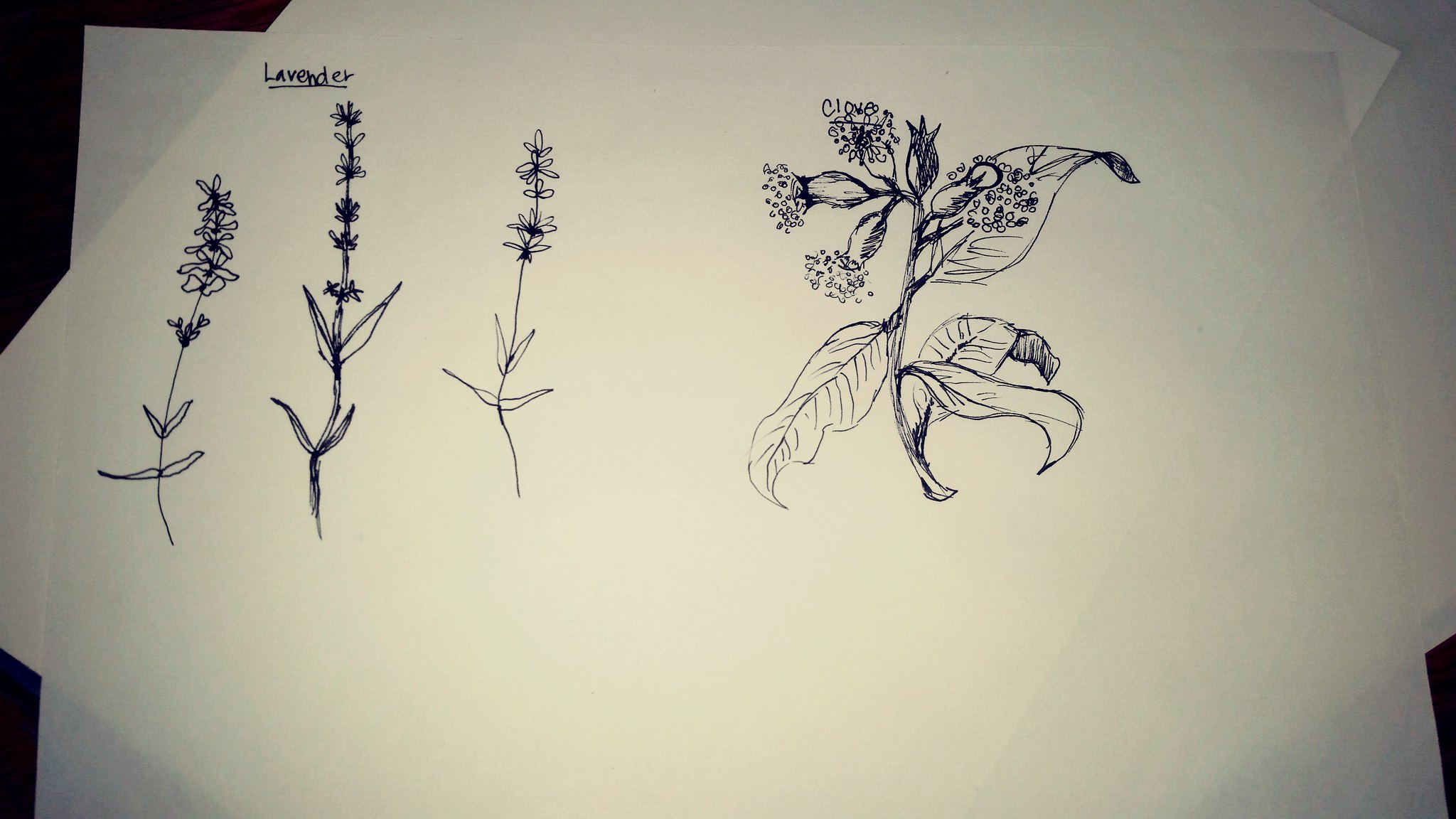This black and white photograph, oriented horizontally, showcases a botanical illustration on a large rectangular piece of tracing paper. The artwork features meticulous black ink sketches of plant specimens. On the left side, the background is predominantly white with small sections of darkened corners. The word "lavender," underlined and written in black ink, labels three vertical sketches of lavender sprigs, each displaying a single bloom. To the right, a detailed drawing depicts a clove plant with bulb-shaped flowers and leaves, with the word "clove" inscribed above it in black ink. Beneath this top sheet, two more layers of paper are slightly fanned out, adding depth to the composition, and the entire scene rests on a dark-colored surface. The precise, textbook-like style of the drawings gives the image an educational, botanical feel.